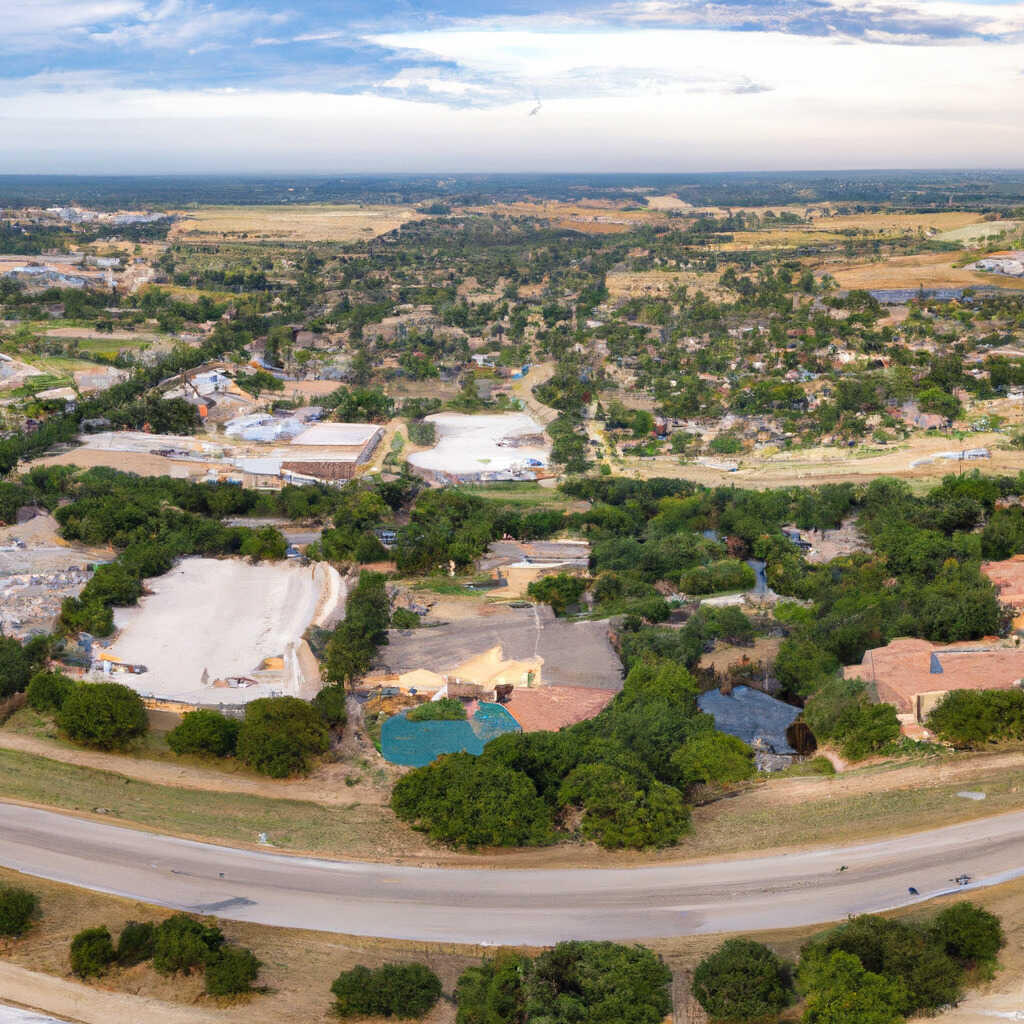This distorted aerial photograph, possibly digitally edited or AI-generated, offers a high-up view resembling that from an aircraft. Looking down, there's a row of trees at the bottom edge, leading to a grassy and dirt area. An ambiguous feature, likely a road rather than water, traverses the scene. Scattered across the midsection are groups of green trees and numerous buildings, with even the presence of parked cars to the left. There are also patches of empty fields and what could be sandy areas. Further back, pools of water, possibly swimming pools, are visible. The overall landscape integrates urban and natural elements, culminating in a distant city skyline. The image, however, appears smudged and irregular, giving it an unreal, painterly quality.